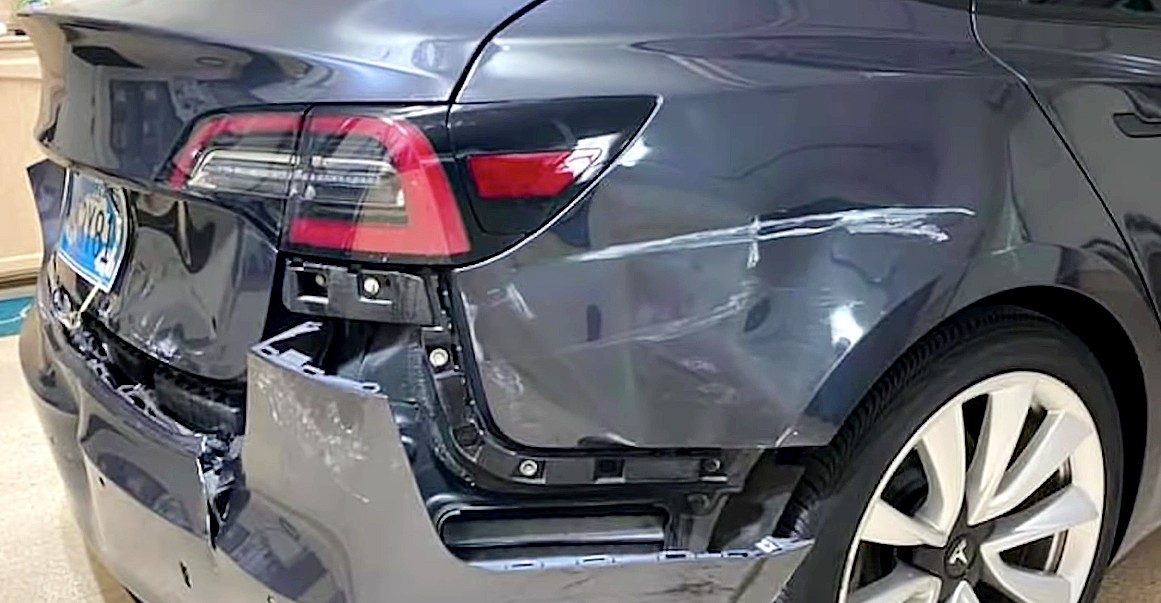This is an image of a dark blue car, likely a small coupe or a Tesla, pictured in a garage, showing significant damage to the back passenger side. The photo focuses on the area where the rear bumper and trunk meet the side fender. The bumper is heavily detached and nearly falling off, with a small black strip with screws visibly disconnected from under the red taillight. There is a large white scratch and a substantial dent on the rear fender area above the rear tire. The tire features an eight-prong silver rim with a visible Tesla logo. The trunk is severely smashed, and a blue and white license plate with black lettering is also visible.